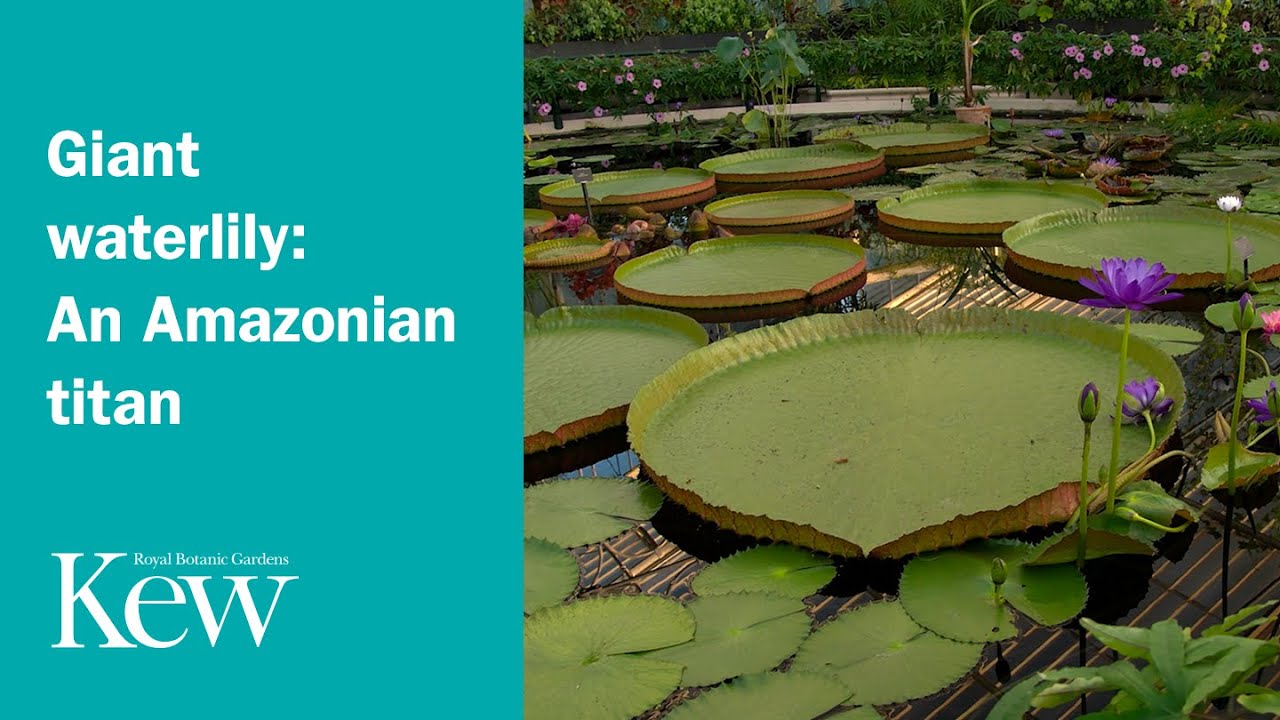The image is an advertisement for the Royal Botanic Gardens, Kew, featuring a striking photorealistic representation of a small garden water enclosure dominated by giant water lilies. On the right side, the water surface showcases a variety of water lilies, including one prominently large lily at the center, punctuated by purple flowers and surrounded by smaller lilies. The water reflects the sky and the Sun, adding a serene quality to the scene. In the background, we observe a trim of bushes with purple blooms, suggesting a well-maintained garden area. The left side of the image is themed with a blue-highlighted background and contains text in white font that reads "Giant Water Lily: An Amazonian Titan," followed by "Royal Botanic Gardens, Kew" in smaller font. The encompassing scene hints at a peaceful, enclosed habitat, with a pool edge and hints of fencing and benches, inviting visitors to sit and marvel at the botanical wonders.